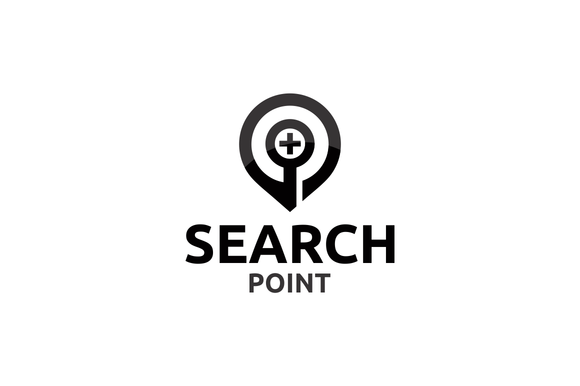The image displays a logo on a plain white background. The logo features a unique combination of shapes: a larger black-outlined circle that partially converges at the bottom, resembling the "you are here" symbol typically seen on maps. Inside this larger circle is a smaller black circle with a black cross in its center, reminiscent of a magnifying glass with a plus symbol. Below the logo, there are two lines of text. The first line, in all caps and black font, reads "SEARCH". Directly beneath it, centered and in a smaller gray font, is the word "POINT". The entire logo appears in a clean black-and-white theme, utilizing a sans serif typeface for the text.